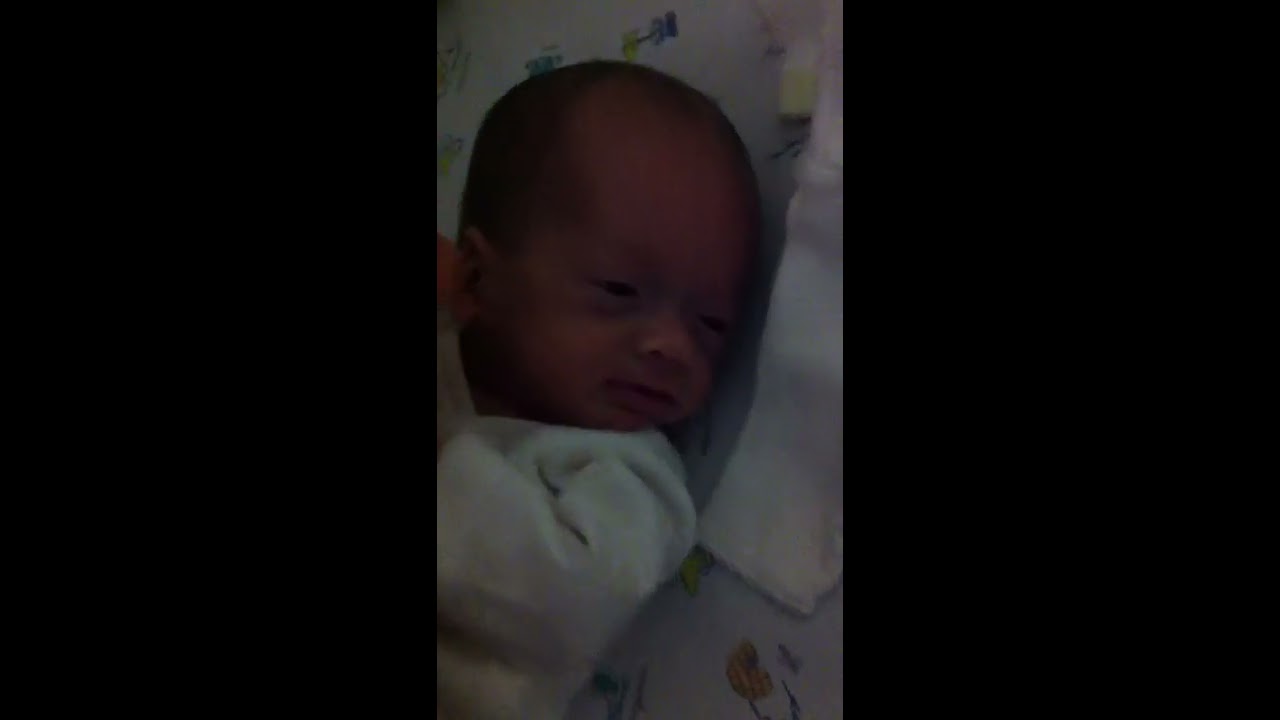This is a horizontally aligned photograph featuring a newborn baby at the center, framed by thick black borders on both sides. The photo has a dark tone due to poor lighting. The infant, with very short patches of black or brown hair, is lying on a patterned sheet that includes colors such as white, green, yellow, blue, purple, tan, orange, and teal. The baby is positioned lying down, head tilted to the left while looking toward the bottom right. The baby is dressed in a white onesie, and only the face, left shoulder, and left arm with the hand up near the ear are visible. There is a white burp cloth placed under the baby's head, with the baby's mouth slightly open, indicating the baby is awake. The photograph appears to be taken indoors, potentially in a crib. No text is visible in the image.